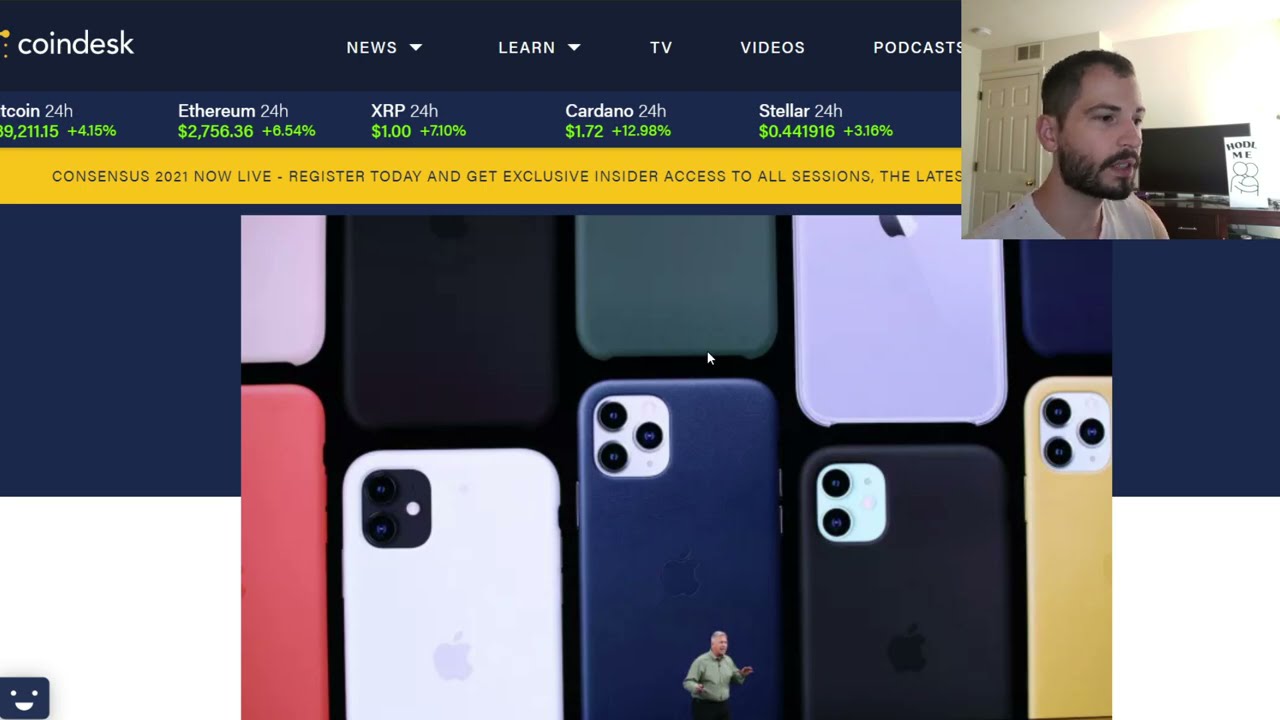The image consists of multiple overlaid elements. In the upper right corner, there is a webcam capture of a white man with a black beard, mustache, and short black hair, dressed in a white t-shirt. He appears to be in a room with a TV and a door behind him, looking off to the right, possibly at a computer screen. The center of the image is dominated by the backs of several smartphones, each adorned with colorful phone covers in shades such as salmon, lavender, white, black, navy, dark green, and light yellow. These phones appear to be Apple devices, distinguished by their varying camera configurations—some have two lenses, while others have three arranged in a triangular layout. Overlaying this scene is a yellow banner that reads, "Consensus 2021, now live. Register today and get exclusive insider access to all sessions." At the very top of the image, the Coindesk logo is prominently displayed, accompanied by cryptocurrency names and their valuation trends, including Ethereum and Stellar. This composite imagery suggests a promotional graphic for a tech event or webcast, likely focusing on phone products and cryptocurrency analysis.